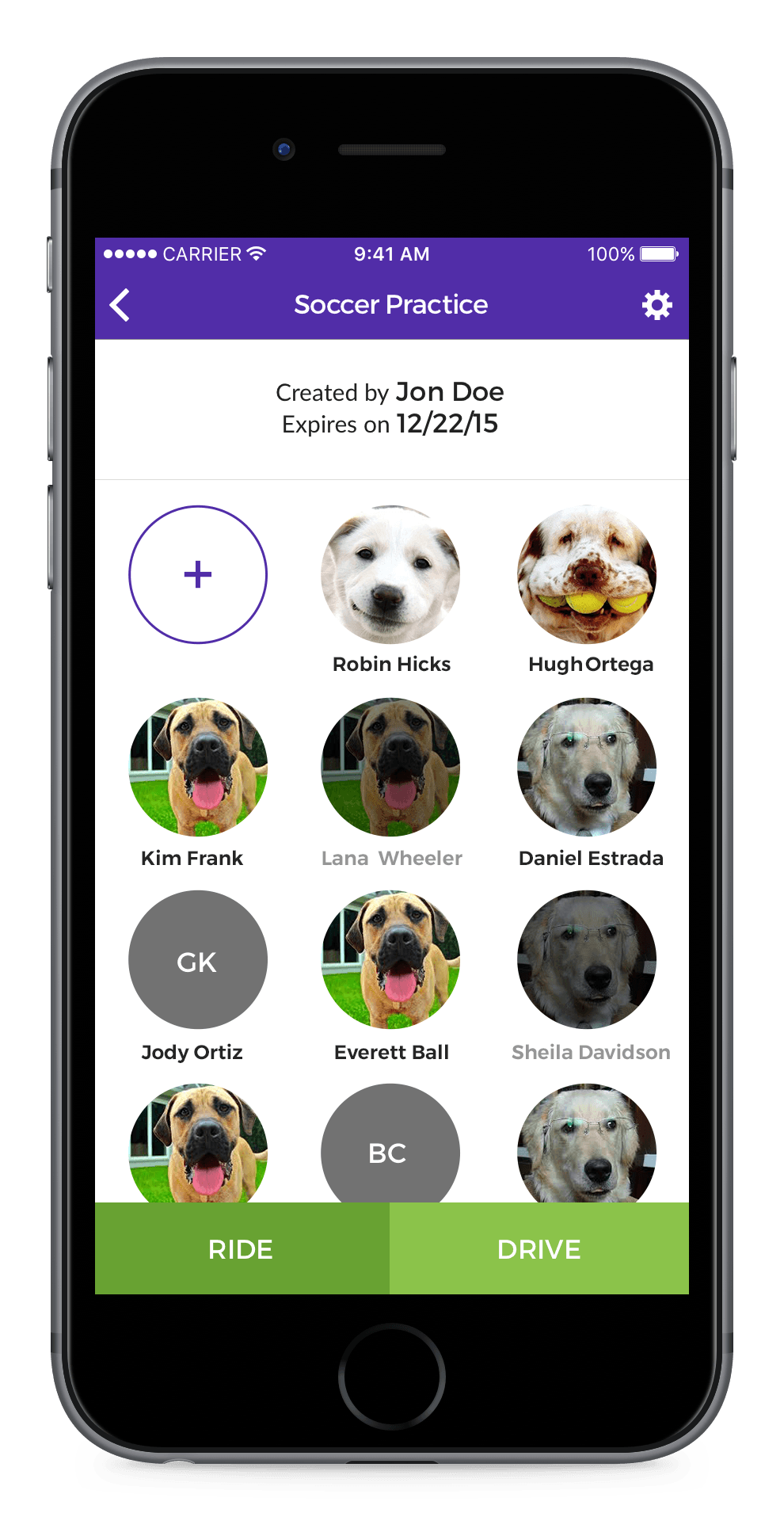The screenshot image is of a digital roster, showing detailed information against a subtle backdrop. At the top center, the current time, "9:41 AM," is displayed, indicating when the screenshot was captured. Below the time, a prominent purple banner reads "Soccer Practice." Beneath the banner, there is a subtext mentioning "created by John Doe" and indicating that the document "expires on 12-22-15." The roster prominently features individual circular photographs of dogs, each associated with names that appear to be human, possibly the owners or handlers. The names listed are Robin Hicks, Hugh Ortega, Daniel Estrada, Kim Frank, Everett Ball, Lana Wheeler, and Sheila Davidson, each name corresponding to a different dog's image in the circles.